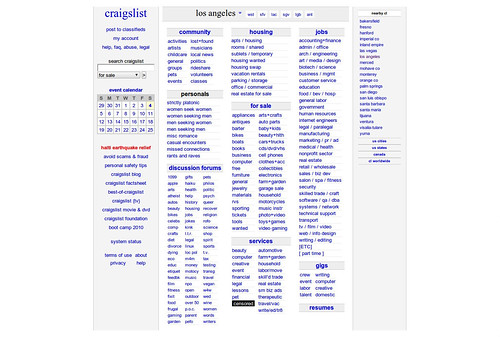This is a detailed screenshot from the Craigslist website. On the left side, approximately two inches in, there's a light gray background strip. At the top of this strip, there is a bold blue "Craigslist" logo. Below the logo, in smaller text, the menu options "Post to Classifieds," "My Account," "Help," "FAQ," "Abuse," and "Legal" are listed in sequence. Following these options, there is a search bar. Directly underneath the search bar is the "For Sale" section header. Progressing further down, the "Event Calendar" link is highlighted in blue, followed by an actual calendar widget. Beneath this calendar, some clickable links are displayed: the first link is in red text, followed by eight links in blue text. A small gap appears before another blue text link, followed by another gap, and then the "Terms of Use," "About," "Privacy," and "Help" links further down.

On the right side of the gray section, there's another light gray area at the top with the label "Los Angeles." Below this label, six small white tabs with blue text are present, though the text is illegible in the screenshot. The background then transitions to white, featuring more blue tabs denoting different categories. The first main category header is "Community" in dark blue text, with seven subcategories listed beneath on the left and seven more on the right. Following this, the categories "Personals," "Discussion Forums," "Housing," "For Sale," "Services," "Jobs," and "Gigs" are listed in black text. 

Adjacent to the main navigation, on the far right side, there is a small white tab with black text that cannot be discerned. Underneath this tab, about 14 blue links, likely subcategories or further navigation options, are listed vertically down the left side. Centered beneath these links are an additional four clickable options, making for a comprehensive and detailed navigation structure of the site.